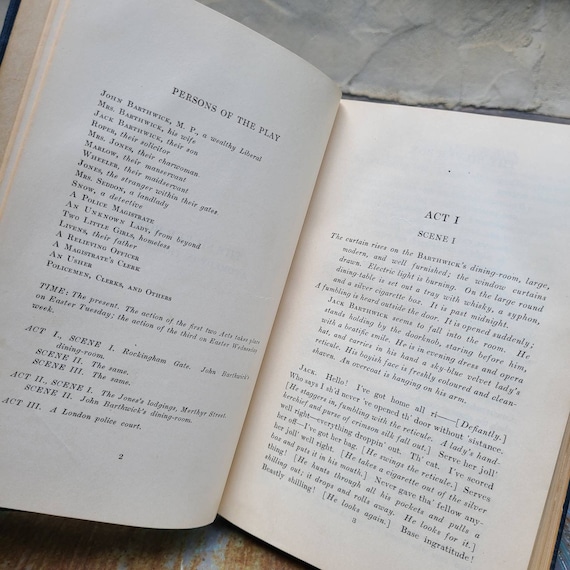The image depicts an open, yellowing playbook resting on a worn and scuffed surface, possibly an old wooden or stone tile floor. The pages are filled with text in English, indicating the play's structure and characters. The left page lists the "Persons of the Play," naming characters such as John Barthwick, Mrs. Barthwick, and Jack Barthwick, among others. The right page details "Act One, Scene One," noting that "the curtain rises on the Barthwick dining room, large, modern, and well-furnished," with drawn window curtains. Above the book, a textured wall serves as the background, enhancing the image's vintage feel. Despite the comprehensive text, the book's title remains unidentified.